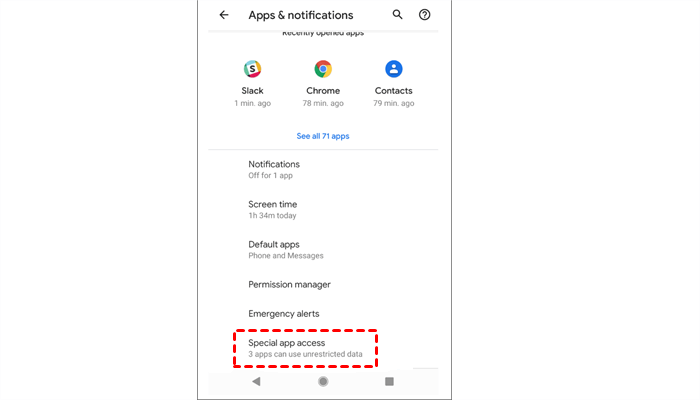This screenshot showcases a smartphone interface with a default black background, presenting a user's notification and app management screen. At the top, there is a white search bar accompanied by a question mark icon and a circular icon to the right, likely indicative of help and additional options respectively. An arrow pointing to the left presumably initiates a return to a previous screen.

Below the search bar, notifications are prominently displayed, with notable mentions such as a Slack notification from one minute ago asking "Am I in?", a Chrome notification from 78 minutes ago, and a Contacts notification from 79 minutes ago. Additionally, there is a blue "See all 71 apps" option for viewing all applications installed on the device.

Further down, category sections are outlined, including "Notifications," where there appear to be "Offer for one app" listed twice. The "Screen time" section indicates usage of 1 hour and 34 minutes for the day. Other sections visible are "Default apps," which lists Phone and Messages, "Permission manager," "Emergency alerts," and "Special app access." Noteworthy is the fact that three apps have permission to use unrestricted data.

Significantly, the "Special app access" section is underlined with red dashes forming a rectangle, accentuating its importance or indicating a particular status requiring attention.

At the very bottom of the screen, a light gray bar houses dark gray navigational icons: a triangle pointing left (back), a circle (home), and a square (recent apps), designed for ease of use.

This detailed information encapsulates the organized structure and comprehensive functionality provided within the smartphone's app and notification management interface.